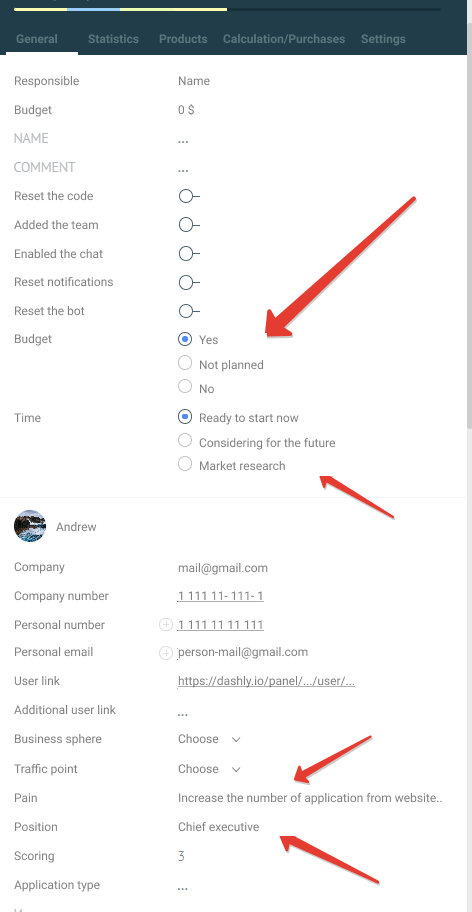A screenshot, seemingly from a phone or tablet, features a dark blue bar at the top with several clickable tabs. In the top left corner, there's a thin line in bright yellow and blue. Below the bar is a two-column layout with numerous single words listed on the left side. On the right side, there are circles, some of which are marked with blue dots, indicating selections.

Key elements include:
- Two red arrows pointing towards the bottom. One highlights a circle marked "Yes" with a blue dot, and the other points to a circle labeled "Ready to start now," also marked with a blue dot.
- A light gray line separates segments as the two-column layout continues downward.
- In the upper left, a circular icon with a picture and the name "Andrew" is visible.
- More single-word options are listed below, with corresponding information filled in on the right side.
- At the very bottom, there are phrases like "Increase the number of applications from the website" and "Chief Executive," both highlighted by long red arrows.

The screenshot appears to be a detailed interface displaying options and selections, possibly from a form or survey.